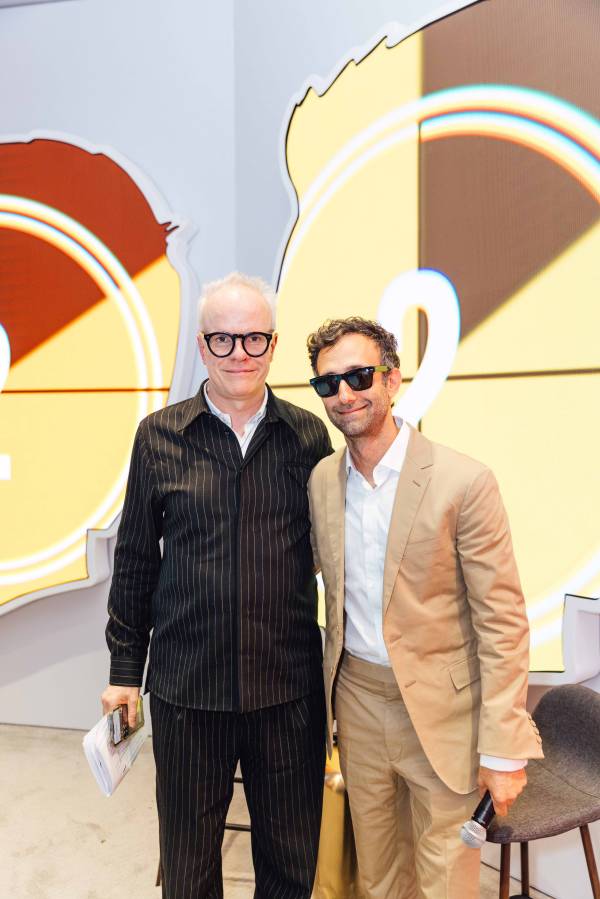In the photo, there are two men standing closely together, appearing to pose for the camera. The man on the left is older, with some graying hair and slight balding, wearing black eyeglasses. He is dressed in a dark brown and white striped blazer with matching pants. His right hand is holding a piece of paper by his side. The man on the right, who has short curly brown hair, is smiling broadly and appears to have his right arm wrapped around the waist of the man on the left, suggesting a warm, friendly connection. He is wearing a tan sports coat over a white dress shirt with matching tan pants. In his left hand, he holds a black microphone and he is also sporting dark sunglasses. Behind them, the background features light blue-gray walls with large circular designs that resemble countdown timers, possibly indicating an upcoming segment. Each circle contains smaller white and red circles with red lines crossing through the center, surrounded by sections of dark gray and yellowish-white colors. There are barstools and a small black chair visible to the right of the men, adding to the scene. The overall atmosphere suggests they are at an event or preparing for a presentation, with both men looking excited and engaged.